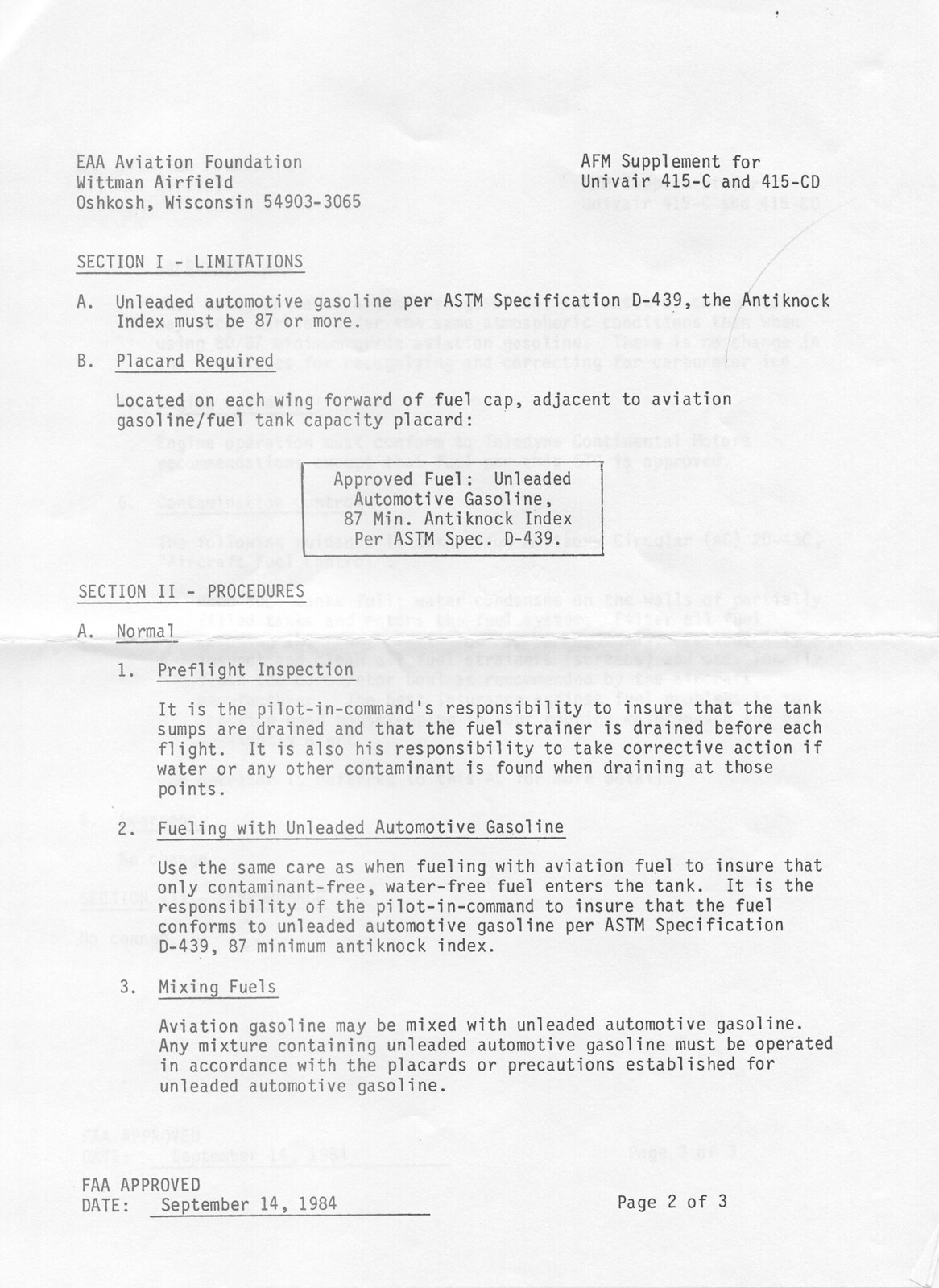The image depicts a black-and-white typed document titled "AFM Supplement for Univair 415-C and 415-CD," associated with the EAA Aviation Foundation at Whitman Airfield in Oshkosh, Wisconsin, zip code 54903-3065. This is page 2 of 3 of the document, which is dated September 14, 1984, and FAA approved. The document is organized into sections detailing aircraft fueling procedures and limitations. Section 1, titled "Limitations," specifies the approved fuel type and the required placard on each wing indicating this type, with an emphasis on using gasoline with a minimum anti-knock index of 87, per ASTM specification D-IV-439. Section 2, titled "Procedures," includes sub-headings such as normal pre-flight inspection (A-1), fueling with unleaded unmetered gasoline (A-2), and mixing fuels (A-3). The text appears in light brown on a white background.